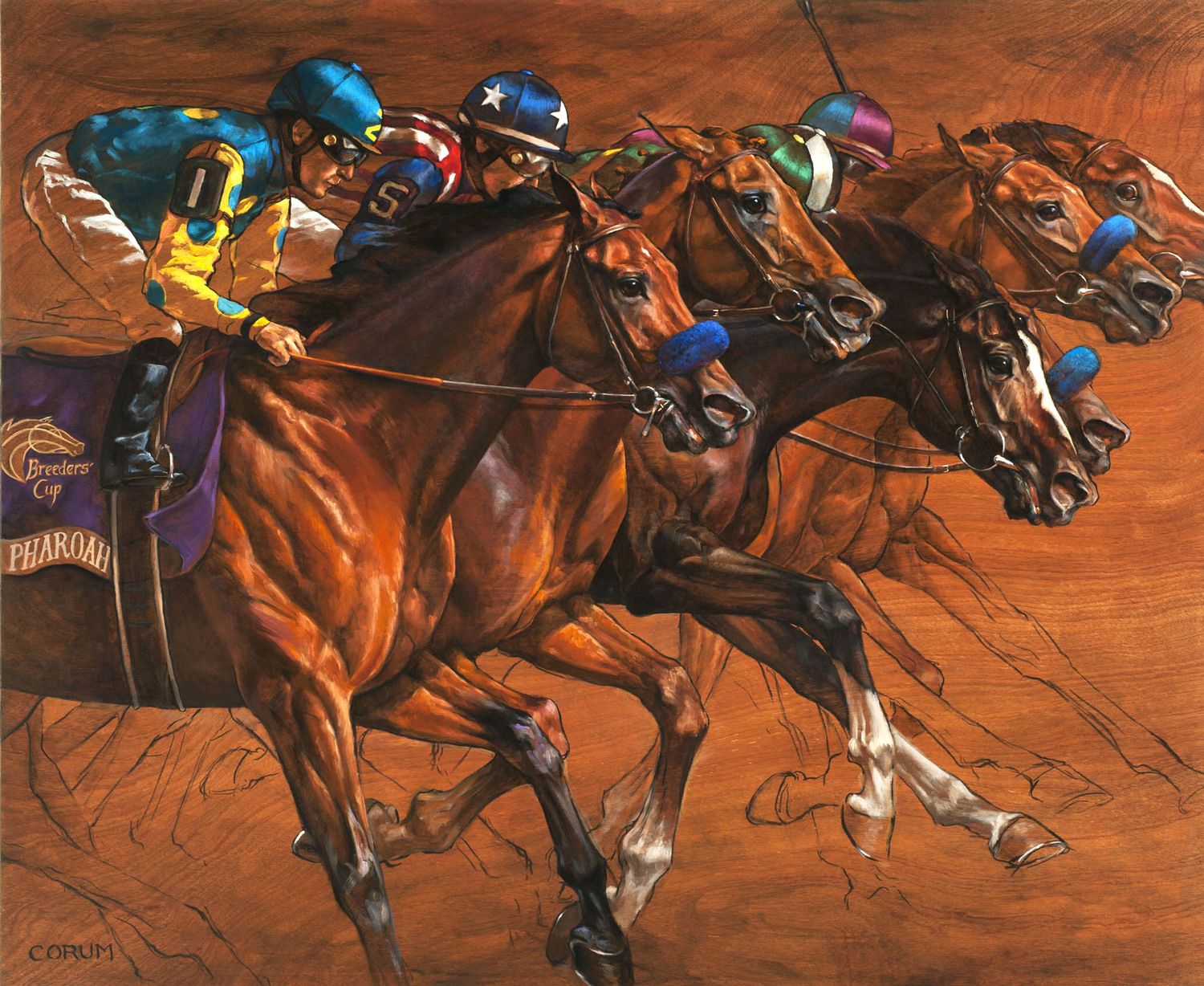This illustration depicts an intense horse race with five hyper-realistic, brown horses, each adorned with black and white accents. The racehorses, sporting various shades of brown, exhibit dynamic motion, enhanced by partially colored sketches of their legs conveying swift movement. Among the jockeys, the first stands out in a teal riding hat and teal-and-yellow shirt paired with light brown pants, riding a horse marked with "Breeders' Cup Pharaoh" on a dark blue saddle blanket. Another jockey features a vivid red, white, and blue outfit with white stars on a blue hat and red and white stripes, distinguished by an 'S' on his sleeve. Other jockeys can be discerned by their colorful hats: green and white, blue and purple. Several horses wear blue nose harnesses linked to the reins held by their jockeys. The untextured, coppery brown background, accented with black smudges, frames the thrilling scene, underscored by the black text "CORUM" at the bottom left.